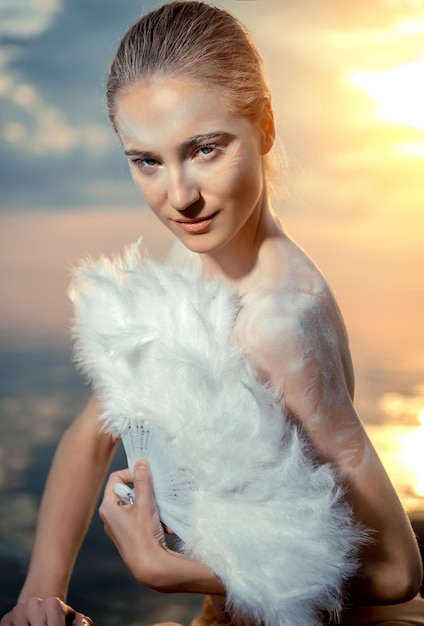This photograph features a Caucasian woman with brownish-blonde hair pulled back, highlighted with white. She leans toward the camera with an almost coy expression, her blue eyes looking directly ahead with her mouth closed. Her skin is layered with a powdery white substance, extending over her face and shoulders. She holds a delicate white feathery fan covering her torso, while her right elbow is bent and pressing down, making her posture appear somewhat awkward.

In the background, a blurry ocean scene is depicted. The left part of the water is a rich blue, transitioning into a striking orange-yellow hue on the right. Above this, the sky mirrors the ocean’s tones with a captivating orange-pink gradient that intensifies with a burst of white in the top right, indicating the sun at sunset. Some puffy white clouds linger in the top left corner, adding further texture to the scene. The interplay of light casts a soft halo effect around the woman, reminiscent of the golden hour, enhancing the ethereal quality of the photograph.